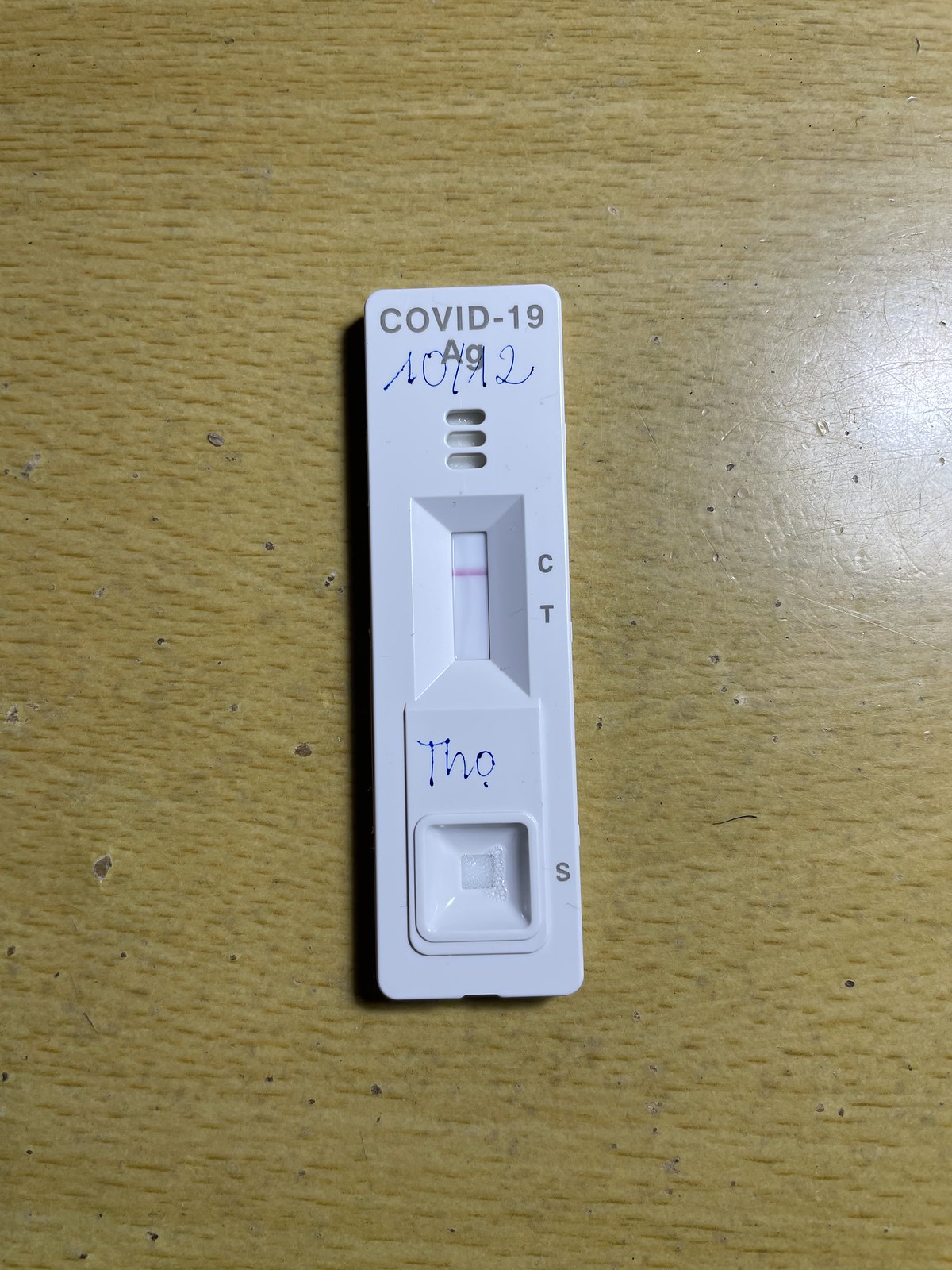The image depicts a COVID-19 antigen (AG) test strip made of white plastic. Prominently displayed on the strip are the designations "COVID-19 AG" with a large "A" and a small "G." Also present is the numbering "10/12" in European style, indicating the manufacture or batch date. On the plastic strip, there are labeled letters "C" and "T" printed in green, alongside a litmus-like paper strip. A dark band on this litmus paper aligns with the "C" position, often signifying a control line. There is also a small cup, likely for sample collection, marked with the letter "S." Additionally, the strip features a handwritten mark that reads "THO," with a period under the "O," written in blue Sharpie ink. All of these items rest on a cream or light brown tabletop, providing a neutral background to the detailed elements of the test strip.